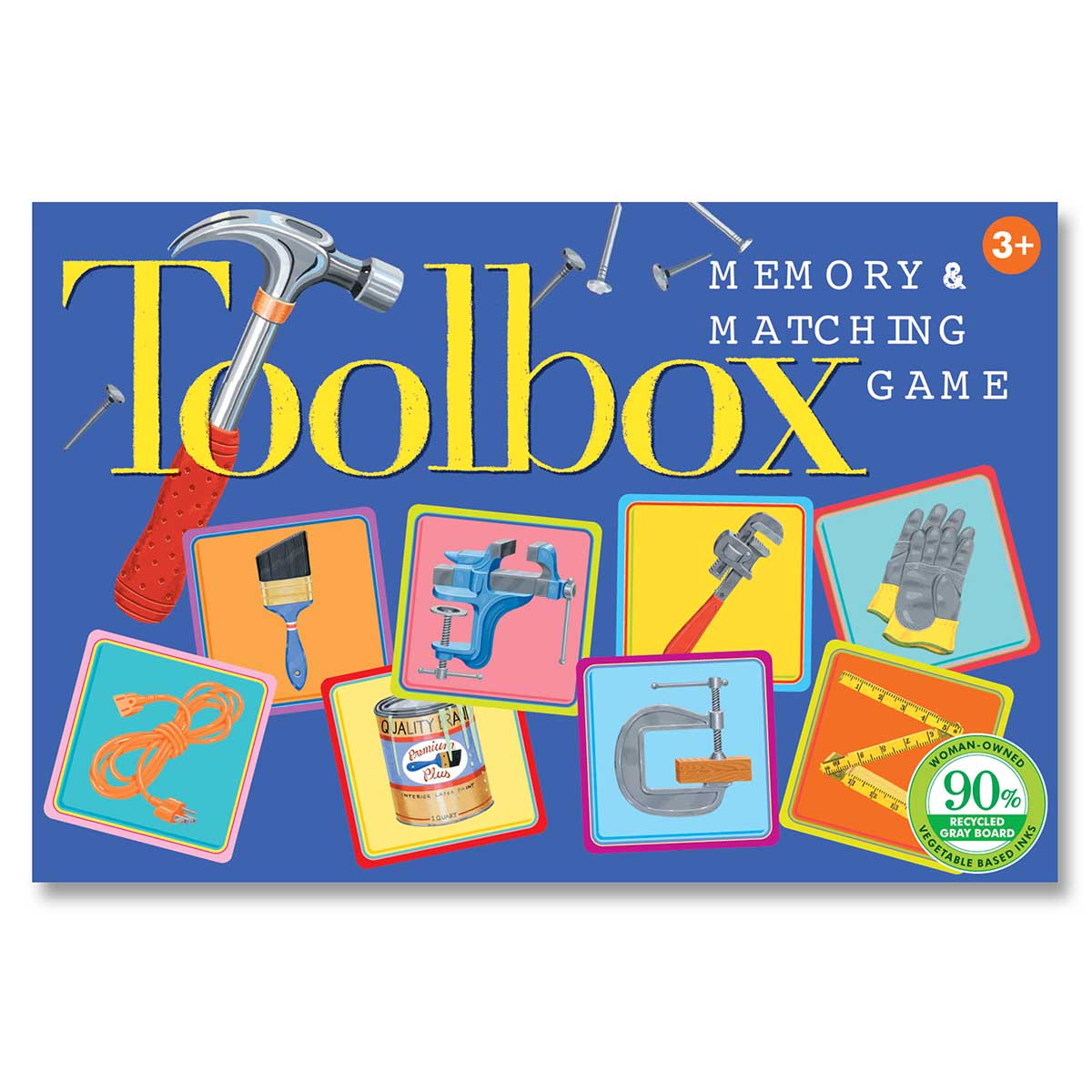The image depicts the cover of a board game box with an ocean blue background. Prominently at the top, the word "Toolbox" is written in bold yellow letters, with a claw hammer creatively integrated into the first "O," protruding outwards. To the right of "Toolbox," in smaller capital letters, it states "MEMORY AND MATCHING GAME." In the top right corner, there's a circular icon with "3+" inside, signifying the appropriate age for the game. Surrounding the word "Toolbox," there are multiple layers adding depth to the design. Below these elements are eight small images arranged meticulously. On the top left is a brush, followed by a blue tool, an orange and grey tool, and a pair of grey and yellow gloves on the top row. The bottom row includes a coil of orange string or wire, a can of paint, a C-shaped tool, and a bendable yellow ruler. The cover is detailed with additional information in the bottom right corner, noting that the game is "Woman-Owned," made from "90% Recycled Grayboard," and printed with "Vegetable-Based Inks." The color palette features vibrant red, orange, yellow, blue, turquoise, black, white, silver, and beige hues, enhancing the illustrative style and playful theme of the board game cover.